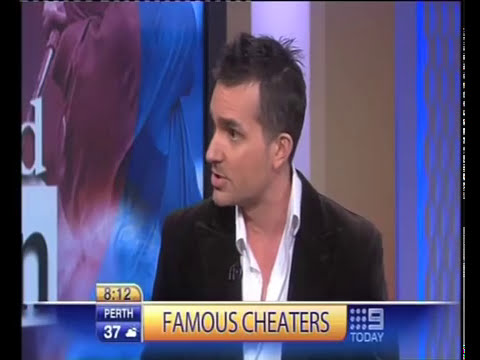The image shows a screenshot from a television show prominently titled "FAMOUS CHEATERS" in bold blue capital letters, encased in a yellow rectangle at the bottom of the screen. Central to the image is a man with short, spiky dark hair, dressed in a black suit jacket over an unbuttoned white shirt, revealing part of his chest. He is equipped with a small microphone on the right side of his jacket. The man, appearing defensive, is looking to his right. 

In the upper segment of the screen, several details are visible: the time "8:12," the location "Perth," the temperature "37°" indicating it's cloudy, and the text "9 today," likely referencing the channel. The backdrop features a studio setting with purplish and bluish hues intermixed with white, brown, and blue stripes, along with mesh detailing. Vertical black stripes frame the outer border of the image. The scene suggests a news broadcast or a talk show, similar to shows like Jerry Springer, with the man seemingly responding to accusations related to the show's theme.